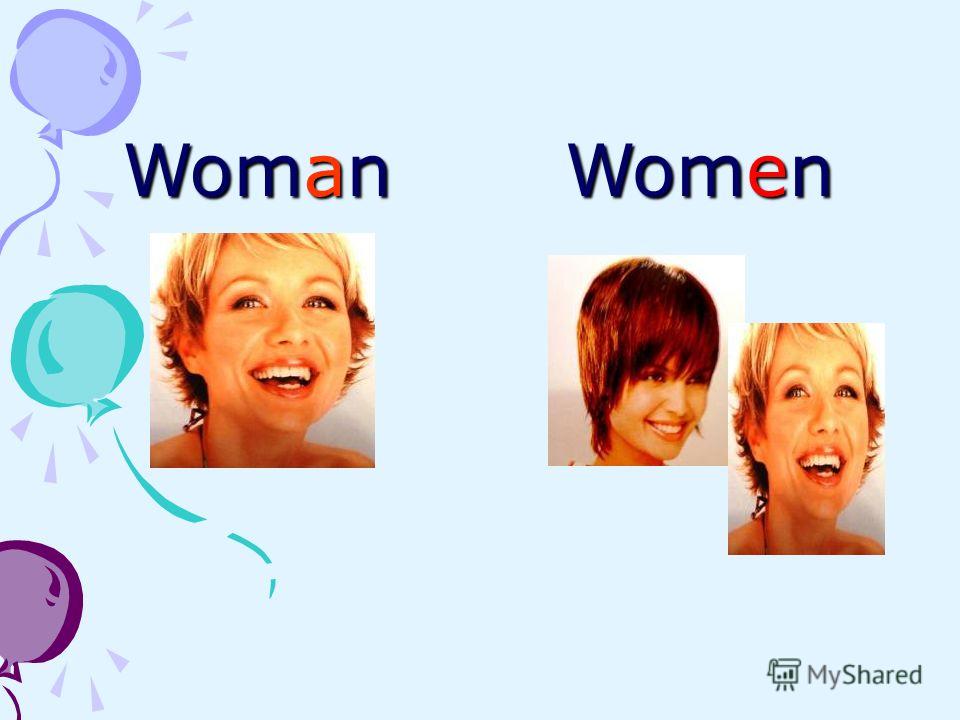The poster uses a light baby blue background to teach the difference between the words "woman" and "women." On the left side, there are three vertically arranged clipart-style balloons in purple, aqua, and light purple (fuchsia), each with three purple arrows pointing at them. Adjacent to the balloons is the singular "woman," written in blue with the letter 'A' in red, above a photograph of a smiling blonde woman with short hair. On the right side is the plural "women," written in blue with the letter 'E' in red, above a photograph of two women. One of them is the same blonde woman from the left, and the other woman has short reddish-brown hair, both smiling. In the bottom right corner of the poster, there is a small graph and the text "My Shared," with "My" in gray and "Shared" in green.